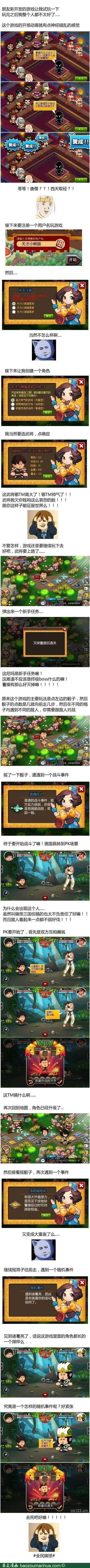This is a very narrow, vertically long image, composed of around 27-28 small, square or rectangular panels arranged in a single continuous strip. Each panel features tiny, detailed drawings in an anime or video game art style, displaying a vibrant mix of colors such as blues, greens, yellows, neon hues, and some browns. The images depict various characters, including men and women, amidst a spectrum of lively scenes. Separating these colored panels are thin white boxes containing text and occasional icons. However, the details are nearly indistinguishable due to the minute size of the panels, making both the intricate images and the text hard to discern, even when zoomed in. The text appears to contain Mandarin writing, lending a cultural context to the strip.